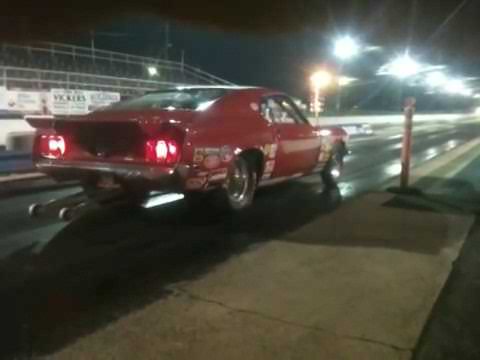The image is a nighttime outdoor scene at a brightly lit racetrack. A vintage, modified red sports car, likely a 1970 Mustang, is positioned on the drag strip. The car is notable for its giant slick black tires at the back, thin black tires at the front, chrome rims on all wheels, a tail spoiler, and numerous stickers on both the front and rear fenders, indicating various auto parts brands. It has a wheelie bar extending from the back, and its two red taillights are prominently visible. The racetrack, bordered by a concrete median with an orange construction barrier, is empty with no spectators in the stands, which can be seen off to the left of the car. The sky is pitch black, but strong overhead lights create a starburst effect, illuminating the scene. The car appears to be poised for a drag race, with the yellow light indicating it's about to start. The entire image exudes an intense, anticipatory energy, with the red car as the focal point against the stark contrast of the nighttime setting.